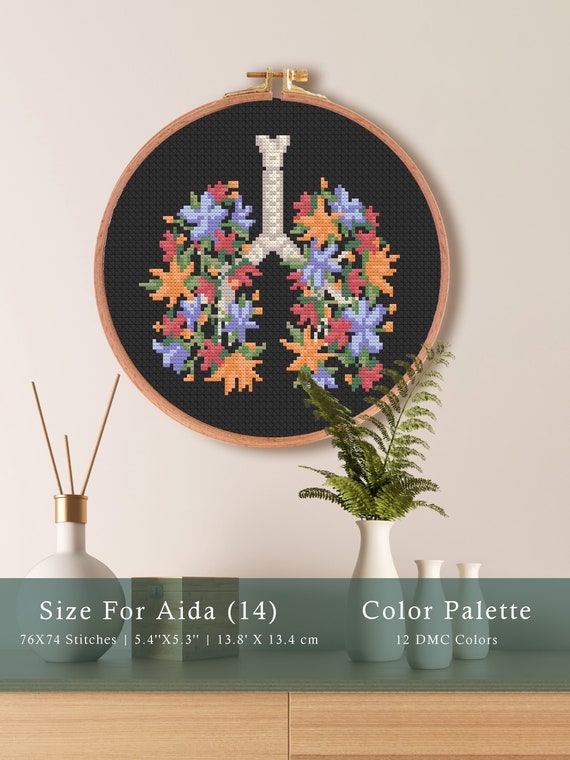The photograph captures a wall-mounted artwork against a dark charcoal gray or black background, displaying a detailed stitch design or embroidery. The focal point of the art is a pixelated tree branch adorned with lavender, orange, and red flowers, positioned as if growing from both edges of the branch. The artwork is framed and hangs from a white wall. Below this captivating piece, a wooden shelf holds a spherical vase containing incense sticks and three cream-colored vases, one with green herbs or ferns. A small wooden box can be seen to the right of one of the cream vases. Additionally, there is a transparent layer over the artwork, indicating specifications: "Size for AIDA 14," with dimensions of 76 by 74 stitches and measurements of 5.4 inches by 5.3 inches, made with 12 DMC colors.